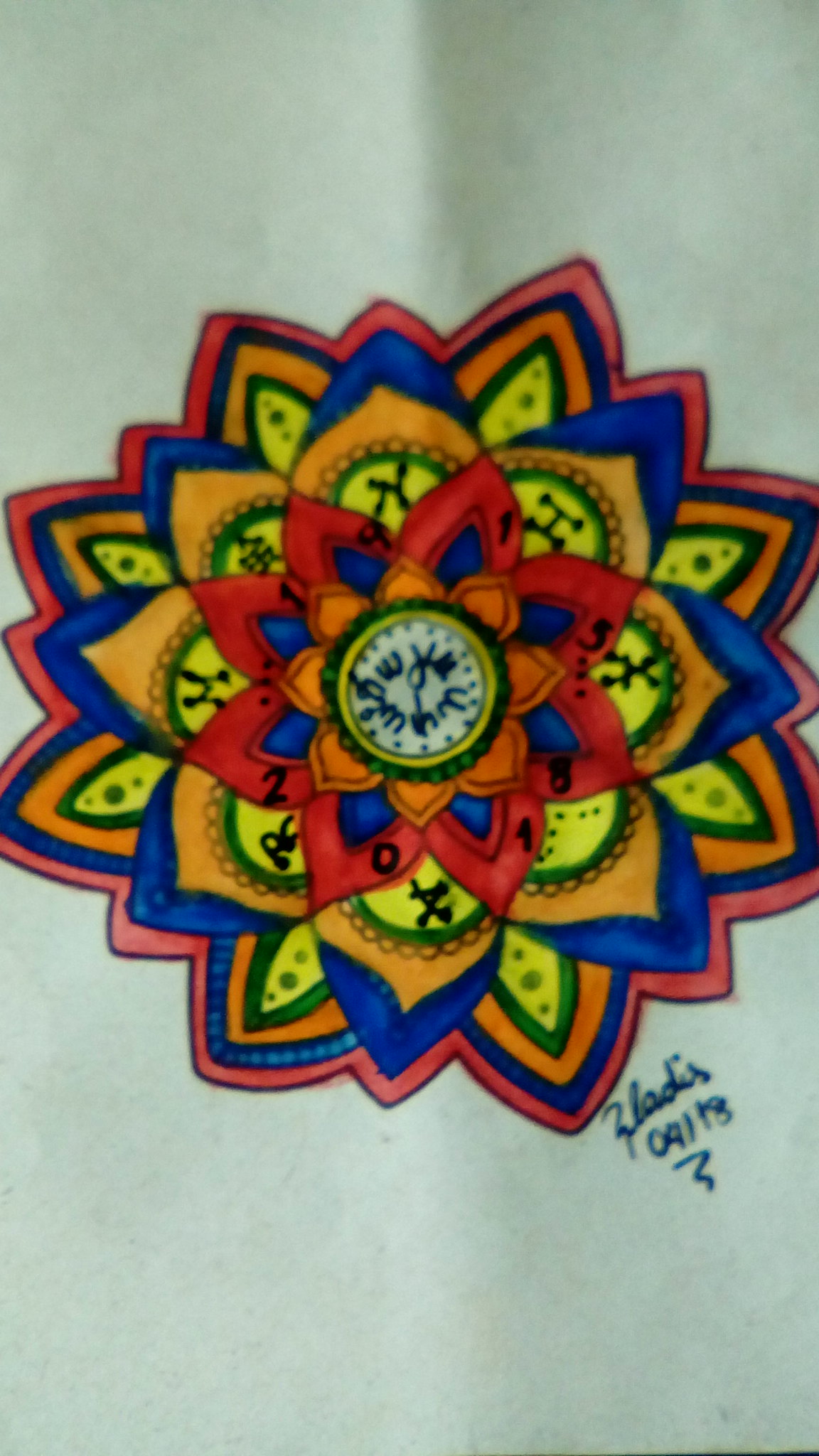This is a detailed color drawing that resembles a mandala of a flower, executed with what appears to be markers on a white piece of paper. The artist's signature, located in the bottom right corner, is written in cursive and spells out "Z-L-A-D-I-S 0918" with a question mark or a squiggly line underneath it, suggesting the date might be April 2018. The intricate flower design consists of multiple layers of petals, each distinct in color: starting from the center, there's a blue section on a white background, followed by a yellow circle with green accents, then a layer of orange petals, succeeded by blue petals, then red petals. The subsequent layers include yellow petals adorned with blue circles, another sequence with blue and orange petals, and ending with green, yellow, orange, blue, and red petals in an alternating fashion. The drawing, though slightly blurry in the photograph, showcases detailed and vibrant coloring.